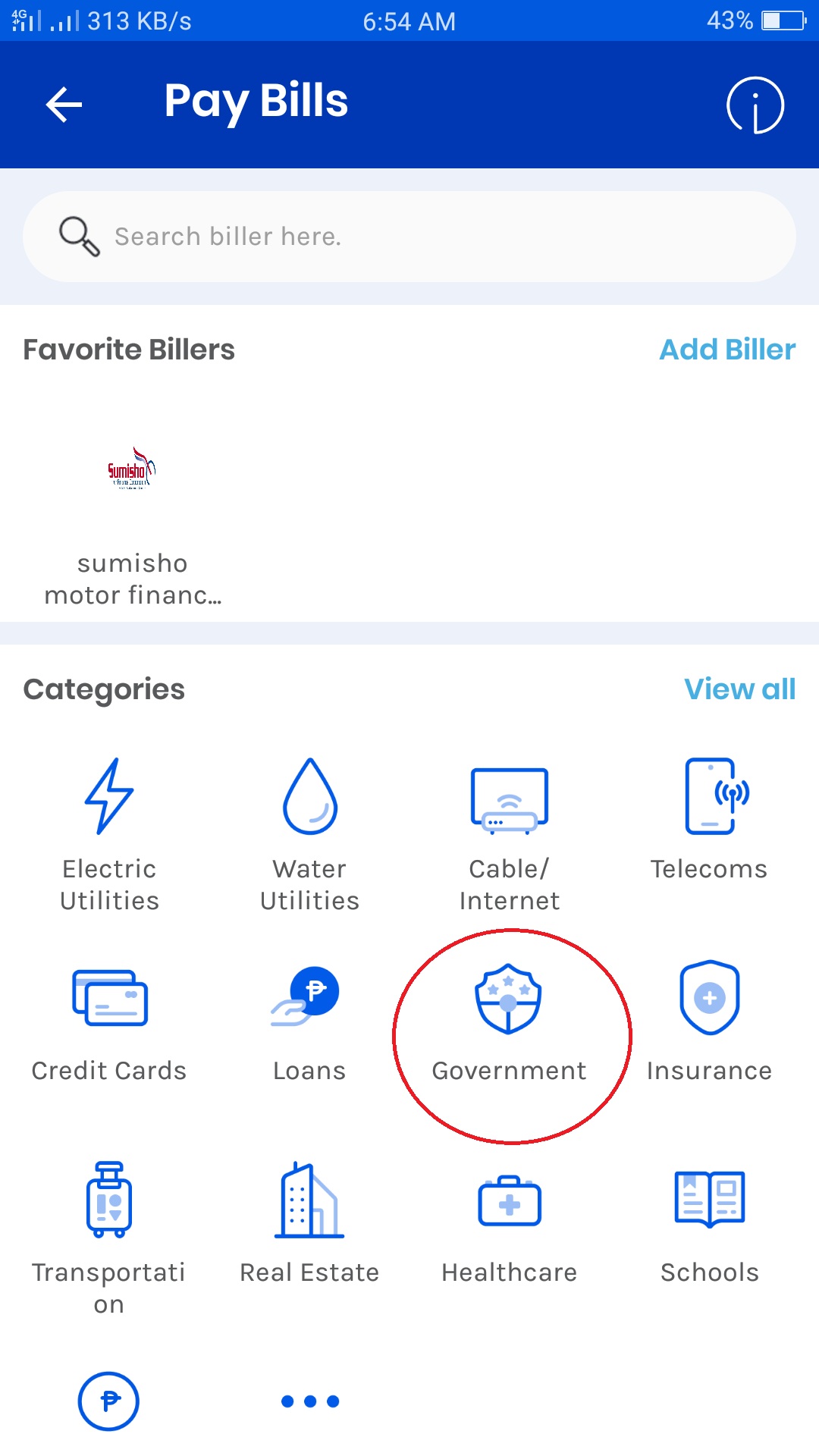The image is a detailed screenshot of a cell phone screen displaying a bill payment app interface. The phone's status bar is customized with a yellow theme and shows various icons including a real-time network connection speed of 313 KB/s, a time display of 6:54 AM, and a battery level of 43%. Below this status bar is a blue header with white text reading "Pay Bills," accompanied by an information button on the right for additional details.

Under the header, there's a search bar for finding different billers. Following the search bar is a section titled "Favorite Billers," featuring "Sumasho Motor Finance," likely indicating the user's car payment service. Below the favorites section, various categories of billers are listed, allowing the user to organize and manage multiple bill payments through the app.

A significant highlight of the screenshot is the "Government" category, circled in red, suggesting its importance in the context of this screenshot, possibly hinting at a tutorial or instructional guide focusing on this category.